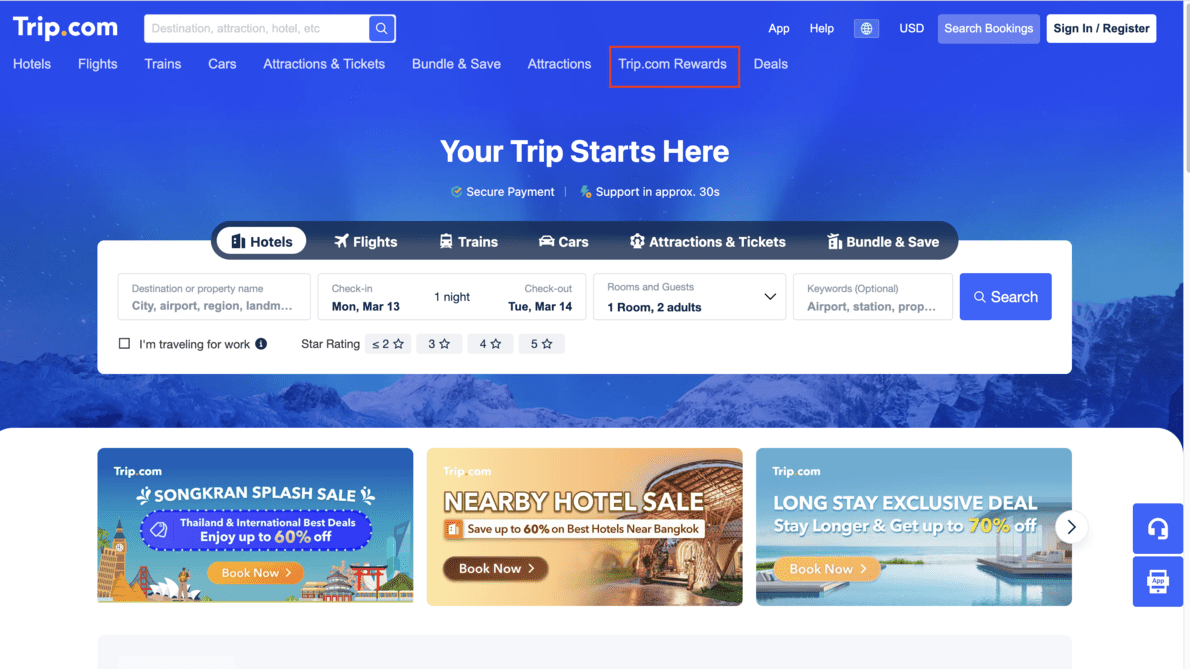The screenshot from the travel website trip.com features a prominently displayed background image in shades of white and blue, depicting scenic snowy mountain ranges. In the top-left corner of the image, the website name "trip.com" is visible next to a search bar. Below the background image, the navigation bar offers various categories such as Hotels, Flights, Trains, Cars, Attractions and Tickets, Bundle and Save, Attractions, Trip.com Rewards (currently highlighted), and Deals. 

In the upper right-hand corner, there are additional navigation options including App, Help, a currency selector labeled USD, a button for Search Bookings, and another button for Sign In or Register. White text beneath the navigation bar proclaims, "Your Trip Starts Here," accompanied by links for Secure Payment and 24/7 Support (noting response in approximately 30 seconds).

A selection banner below this information allows users to choose from options such as Hotels, Flights, Trains, Cars, Attractions and Tickets, and Bundle and Save, with Hotels currently selected. Below this, there is a reservation window for hotels where users can enter check-in and check-out dates, specify the duration of stay, and detail room preferences. On the far right of this window, a large blue "Search" button is visible.

Towards the bottom of the page, a white section displays various savings deals in three banner windows. To the right, two square blue buttons are shown, with the top button featuring an icon representing headphones and a microphone.